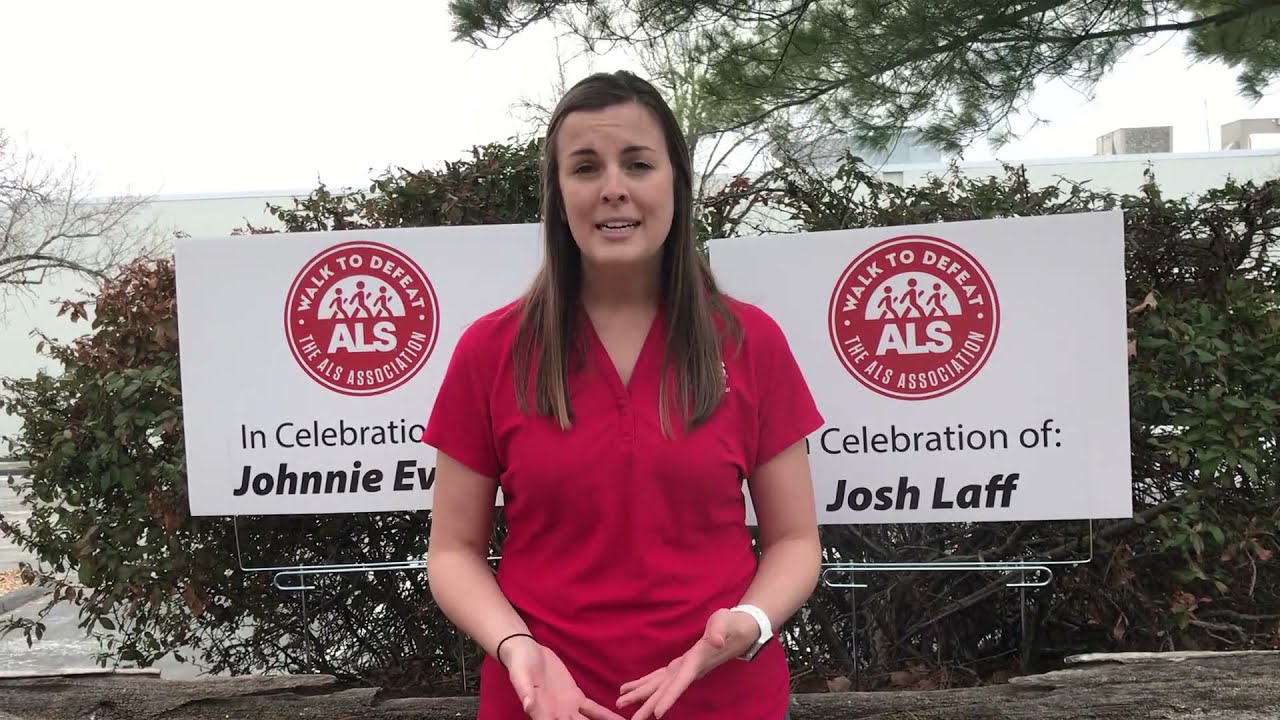In this image, a woman in her early 30s with long brown hair is captured mid-sentence, suggesting it's a still from a video. She is standing outdoors in front of a building partially obscured by trees and bushes. The woman is wearing a red v-neck blouse and red pants, with a white watch on one wrist and a black bracelet on the other. Behind her are two signs with the red logo of the ALS Association that read "Walk to Defeat ALS." The signs also feature names in black text, "In Celebration of Johnny EV" on the left and "In Celebration of Josh Lab" on the right, likely honoring individuals affected by ALS. The overall scene indicates a reporter or presenter discussing a fundraising event related to ALS awareness.